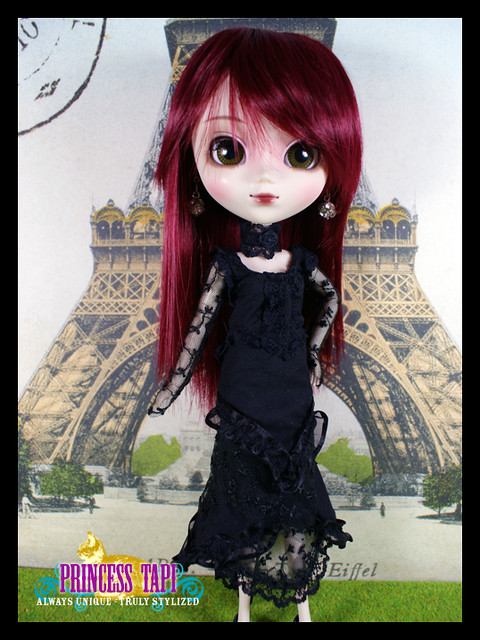This color image showcases a doll named Princess Tapi standing in front of an image of the Eiffel Tower, which appears to be part of a light-colored postcard complete with a stamp in the upper left-hand corner. The doll has an exaggerated, large head with strikingly large brown eyes, a tiny mouth adorned with red lipstick, and exceptionally long cherry red hair. She is dressed in an elegant, very long black dress featuring lace sleeves, lace accents, and a lace bottom, complemented by a black choker necklace. The doll has light skin and Asian features, evoking a young anime girl aesthetic. The background includes small trees and a grassy area. At the bottom left of the image, it reads in purple letters "Princess Tapi, always unique, truly stylized," and at the bottom right, it says "Eiffel."